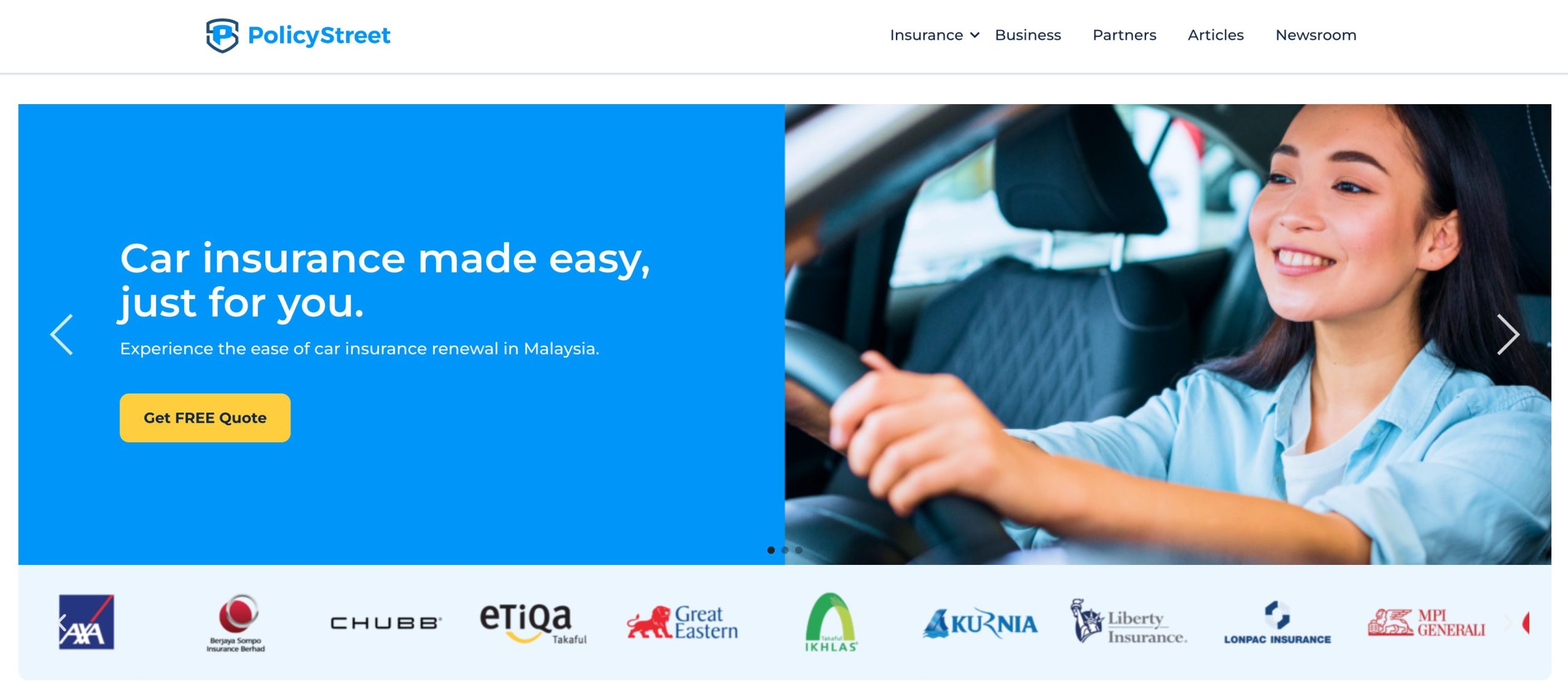A screenshot of a small section of a website captures various elements. At the top left, slightly offset, the words "Policy Street" are displayed in blue, accompanied by a small icon to the left. Moving to the right, there are five navigation options: "Insurance" with a dropdown menu, "Business," "Partners," "Articles," and "Newsroom." A thin gray line spans the width of the section.

Below this line is a blue advertising banner that stretches across the screen. On the left side of the banner, against a solid blue background, white text reads "Car insurance made easy just for you," with smaller text underneath and a yellow "Get a free quote" button. To the left of this text, an arrow suggests the option to scroll between different panels.

The right side of the banner features an image of a woman smiling and holding a steering wheel inside a car. An arrow to the right of this image indicates navigation to the next banner.

At the bottom of the screenshot, a light blue banner lists various company logos. There are ten different logos, although some are too small to identify. Recognizable logos include Chubb, Etiqa, Great Eastern, Liberty Insurance, and MPI Generali. Additionally, each company listing is accompanied by either their logo or advertisement images.